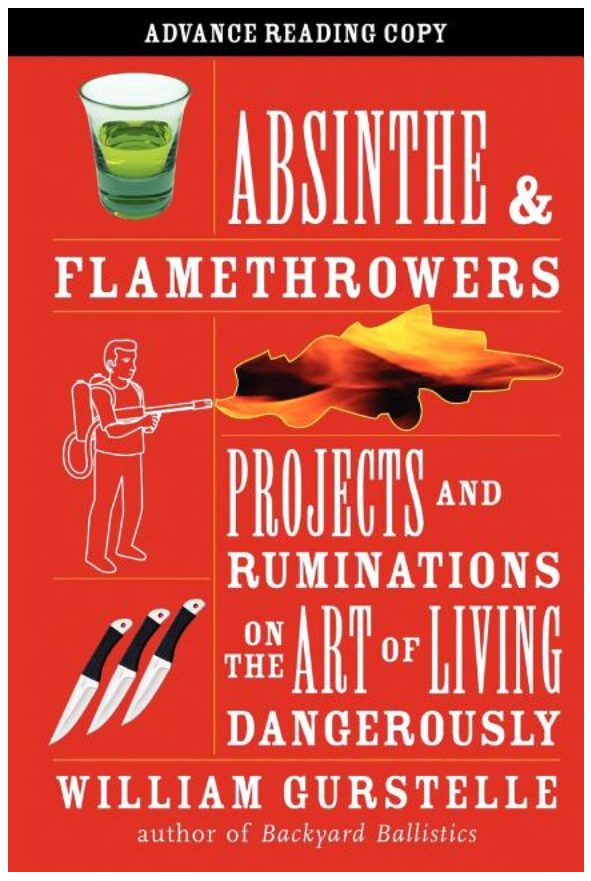This image features an advanced reader's copy of the book titled "Absinthe and Flamethrowers: Projects and Ruminations on the Art of Living Dangerously" by William Gerstel, author of "Backyard Ballistics." The book cover is an all-red background with a distinctive black bar at the top, where the phrase "advanced reading copy" is displayed in white lettering. The title "Absinthe and Flamethrowers" is prominently placed in the center, with a small shot glass of green absinthe illustrated next to the word "Absinthe" at the top. Beneath the word "Flamethrowers," there is a white doodle of a man holding a flamethrower, with stylized orange flames issuing from it. Below this illustration, three different knives or daggers are depicted. The color scheme of the cover includes red, black, white, green, and orange elements, creating a visually striking design.